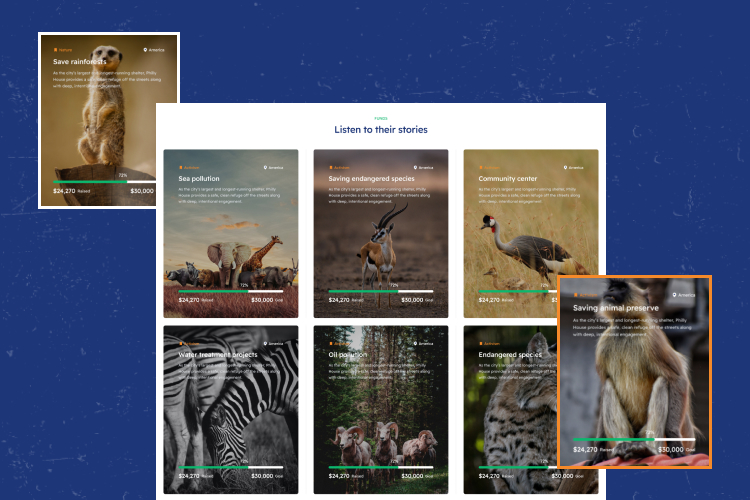The screenshot displays a webpage with a solid blue background. At its center is a large, white square featuring six different photos of animals, each associated with various environmental and conservation messages. The photos are as follows:

1. A meerkat, with text encouraging the viewer to "Save the Rainforest."
2. An elephant, alongside a call to action for "Saving Endangered Species."
3. A community center initiative presented by another image.
4. An image addressing "Endangered Species" impacted by "Oil Pollution," featuring a ram.
5. A zebra, presumably involved in another conservation effort.
6. A monkey, with a message about "Saving Animal Preserve."

The prominent white square also contains the text "Listen to Their Stories" written in blue, unifying the images with a common narrative. Additionally, there is mention of a photograph featuring either a duck, turkey, or goose, included in the awareness campaign. This detailed caption highlights the diverse aspects of the webpage's focus on animal conservation and environmental protection.